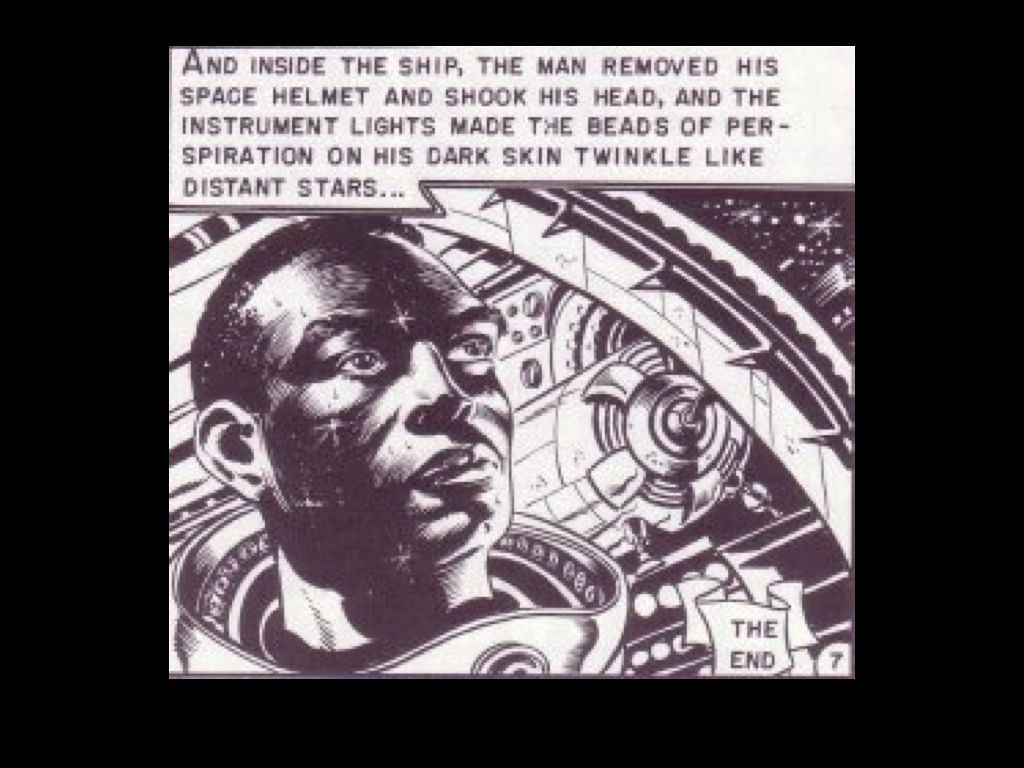In this detailed black-and-white comic strip panel, framed by a thick black border, a short-haired black astronaut is depicted on the left side, gazing out of a spaceship window into the vast expanse of space. The astronaut, dressed in a futuristic space suit with a large collar around his neck, is removing his helmet and shaking his head. The intricate drawing style, likely done with pencil or pen, captures the scene vividly, showcasing the spaceship's machinery around him and the instrument lights within the ship. These lights cause the beads of perspiration on his dark skin to glisten like distant stars, adding to the atmospheric tension of the scene. Above him, a speech bubble narrates, "And inside the ship, the man removed his space helmet and shook his head, and the instrument lights made the beads of perspiration on his dark skin twinkle like distant stars." The panel concludes with the words "The End" in the lower right corner, hinting at the close of an epic space adventure.